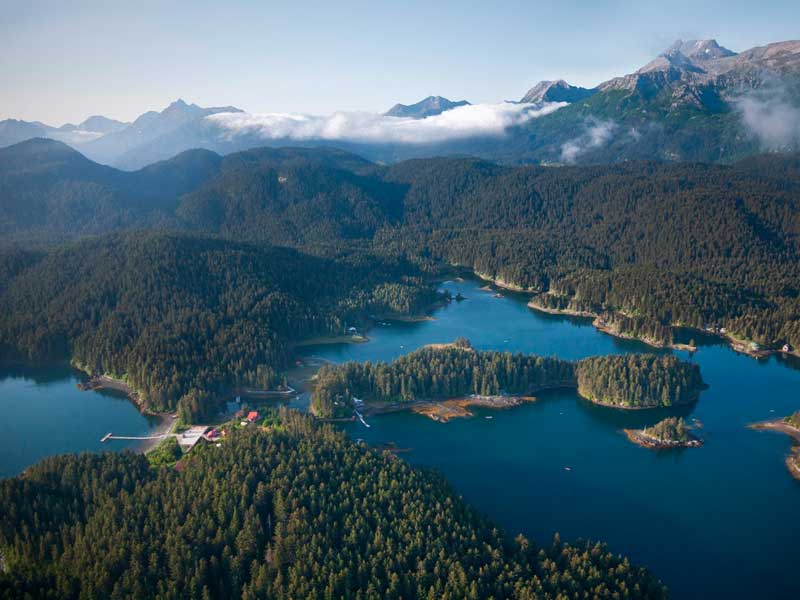This stunning aerial photograph captures a breathtaking vista of a tree-covered mountain region dominated by a large, serene lake. The top of the image features a majestic mountain range with tall, grey peaks piercing through a veil of low-hanging clouds under a pale blue sky. Below the mountains, rolling hills blanketed with dense forests descend towards the expansive lake, which cradles several tree-clad islands within its tranquil waters. 

To the left of the image, at the lake's edge, a pier or dock is visible, accompanied by a structure that could be a house or a business. A few small boats are scattered on the water's surface. The photograph, taken from a high aerial perspective, highlights the natural beauty and intricate details of the landscape, from the shaded hills influenced by varying sunlight, to the man-made elements subtly interspersed within the scene. The presence of buildings or a boat launch suggests a human touch amid the untamed wilderness, adding contrast to the lush, verdant surroundings.